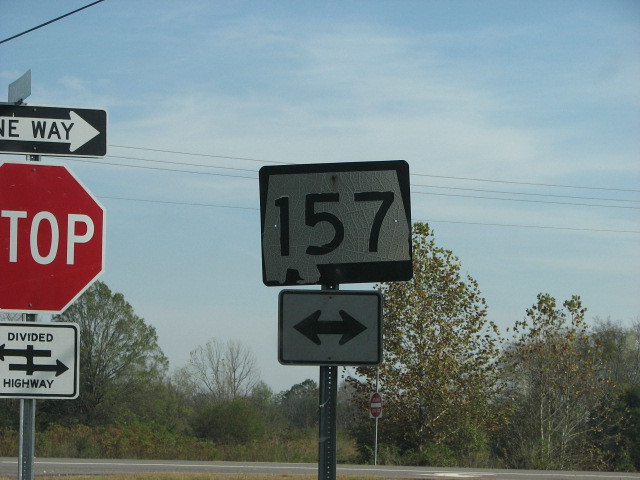In the image, we are presented with a close-up view of several road signs positioned at the side of a highway. Foremost in the image is a series of signs mounted on various poles. Dominating the scene is a black and white one-way sign featuring a white arrow, positioned above a red octagonal stop sign with "STOP" in bold white letters. Below the stop sign is a divided highway sign, characterized by a white background with two black arrows pointing in opposite directions, separated by a line. 

Adjacent to this grouping, on a separate green pole, is a worn highway sign displaying the number 157. This sign is black and white, slightly weathered, and includes an arrow indicating both directions. To the rear of these signs, another pole holds a red and white "Do Not Enter" sign with a white square background. 

In the background of the image, beyond the signs, is a tarmac road marked with white lines, leading towards tall green trees and bushes. Above the trees, power lines stretch across the blue sky, which is adorned with wispy, hazy clouds. The scene, detailed and complex, showcases the various road signs with the natural elements and infrastructure subtly framing them.